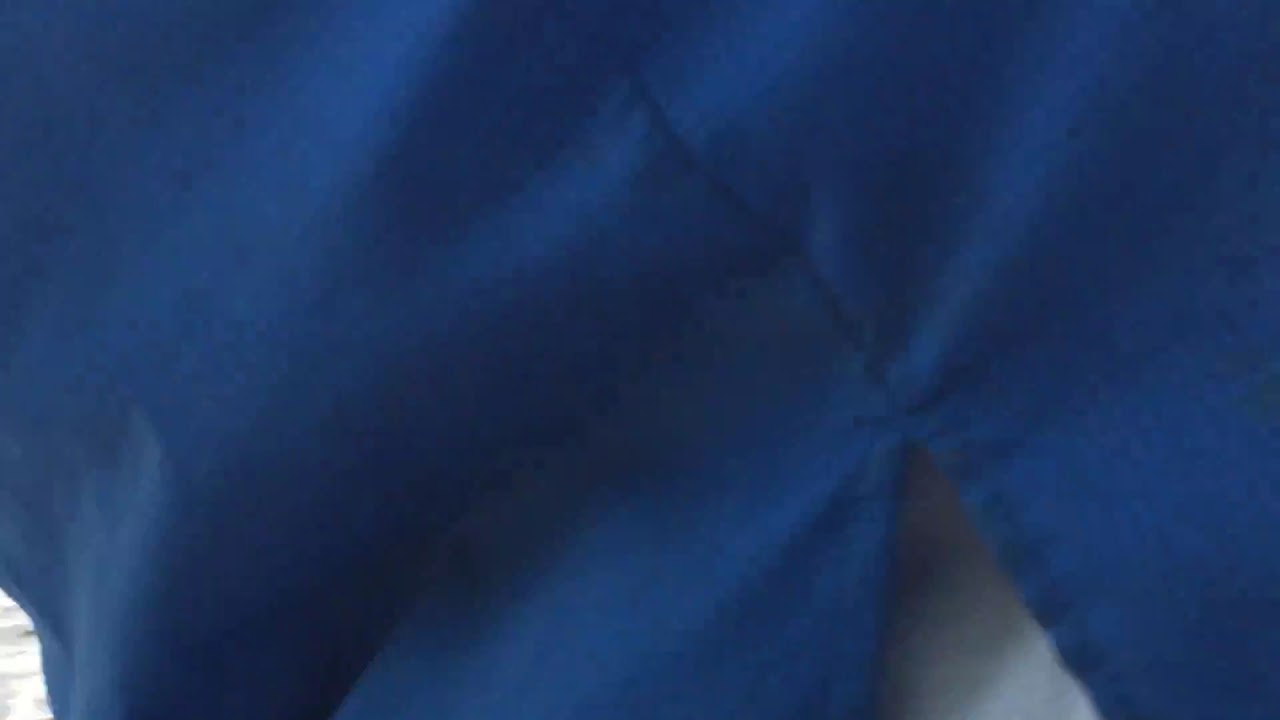The image depicts a close-up view of a dark blue cloth, possibly a pair of pants or the top of a garment, featuring noticeable wrinkles and stitches. Prominently, there is a stitched line running through the cloth, which ends in a triangular V-shaped cut. Behind this cut, a white material can be seen, adding contrast to the blue fabric above. The cloth lies on a flat surface, perhaps a white sheet, arranged in a somewhat wavy pattern. The photograph is rectangular, with its length greater than its width, capturing mostly the blue fabric and its detailed texture.